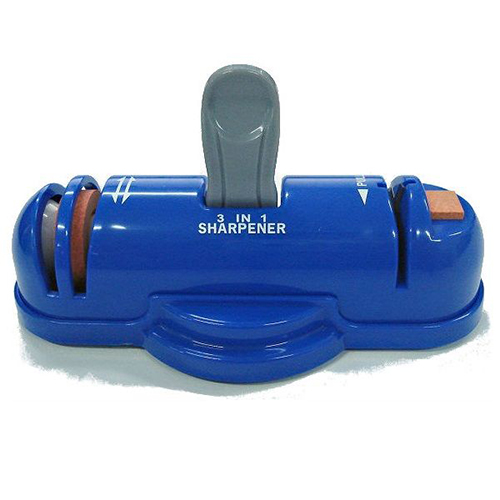The image displays a blue, oblong 3-in-1 knife sharpener against a white background, casting a subtle shadow beneath it. Centered on the sharpener, in white all-caps text, is the label "3-in-1 SHARPENER." The product features three distinct notches: two on the left and one on the right. The left side slots house two sharpeners—a red one and a gray one—possibly designed to accommodate different blade types. In the middle, above the label, is a gray tab resembling a can pull tab, which might be pushed to activate or adjust the sharpening mechanism. The right side has a wider slot with an arrow symbol pointing downward, indicating the direction for use. The notches appear to have buffers, likely for holding and guiding the knives while sharpening. The entire setup suggests it’s a versatile tool for sharpening various kinds of knives with specific instructions to ensure proper usage.